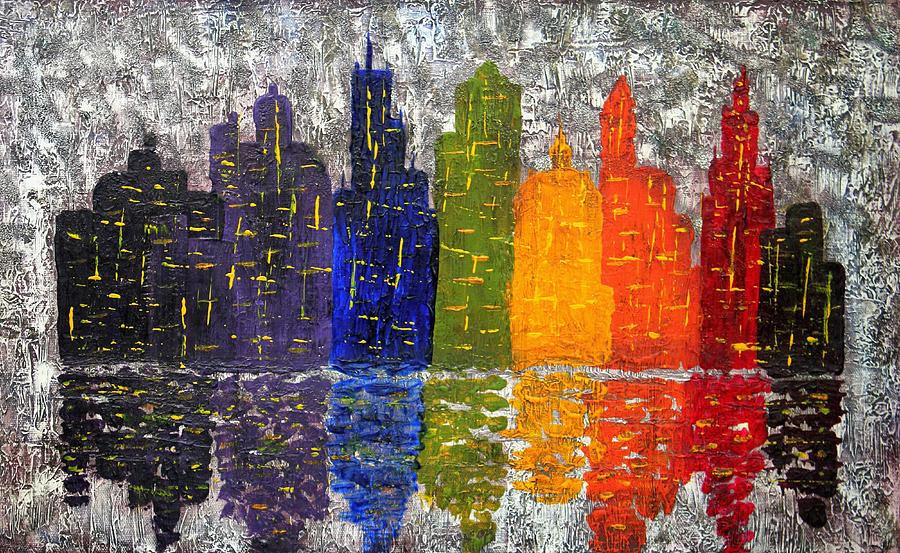The painting depicts an abstract city skyline against a mottled gray background with hints of blue and white, creating a textured, almost palette knife-like effect. The skyline features a series of high-rise buildings painted in a gradient of colors, starting from a black building on the far left, followed by a purple, blue, green, yellow, orange, light red, and dark red building, and ending with another black building on the far right. The buildings have a patchy, smudged texture, suggesting the use of oil paints. Thin streaks of yellow, resembling lights, crisscross horizontally and vertically through the buildings, adding a dynamic element. Below the skyline, a blurry reflection of the buildings can be seen, mirroring the colorful structures, further enhancing the abstract nature of the artwork.